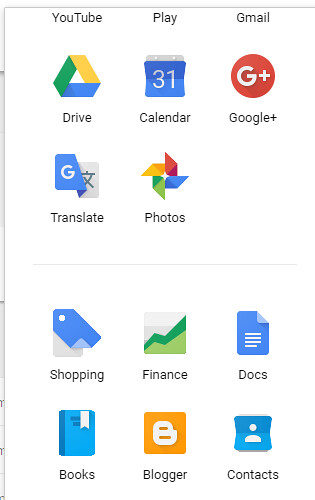The image is a partial screenshot of a phone or computer screen, arranged in a grid layout. It features a gray horizontal line across the middle, which doesn't extend to the edges. The left border is gray with small black dots scattered in various places. The top border is also gray. Just below the top gray border, the words "YouTube," "Play" and "Gmail" are visible. Below this, there's a grid section on a white background.

In this grid, several icons and their corresponding labels are visible:
- The Google Drive symbol labeled "Drive."
- A calendar icon with the number 31 in blue, labeled "Calendar."
- A red circle with a white "G+" symbol, labeled "Google Plus."

In the following row:
- A blue "G" icon in front of a folded rectangle labeled "Translate."
- The Google Photos icon, a colorful symbol in yellow, green, blue, and red, labeled "Photos."

Beneath the horizontal gray line, several more icons are visible, labeled "Shopping," "Finance," "Docs," "Books," "Blogger," and "Contacts."